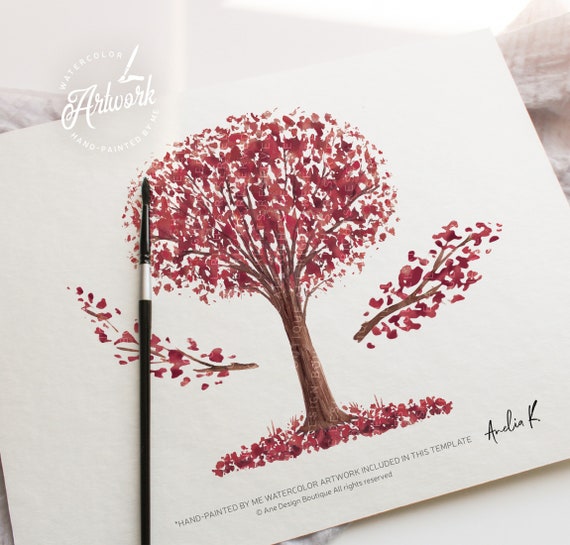This is a promo picture of a watercolor painting by the artist Amelia Kay, prominently featuring a tree adorned with rich, burgundy-red leaves, possibly resembling cherry blossoms in early fall. The tree stands as the central figure with a trunk of deep brown and is surrounded by scattered red leaves on the ground, enhancing the seasonal ambiance. Two artistically cut branches dangle midair, adding an intriguing element to the scene. The painting, relatively small and reminiscent of a stationery card cover, includes a visible watermark at the top that reads, "hand-painted by me, watercolor artwork," and is signed by Amelia Kay herself. The artist's paintbrush rests to the left of the artwork, further grounding the scene in its creative context. At the bottom of the image, additional details indicate, "hand painted by me, watercolor artwork included in this template, copyright and design boutique all rights reserved," completing the professional and aesthetic presentation.